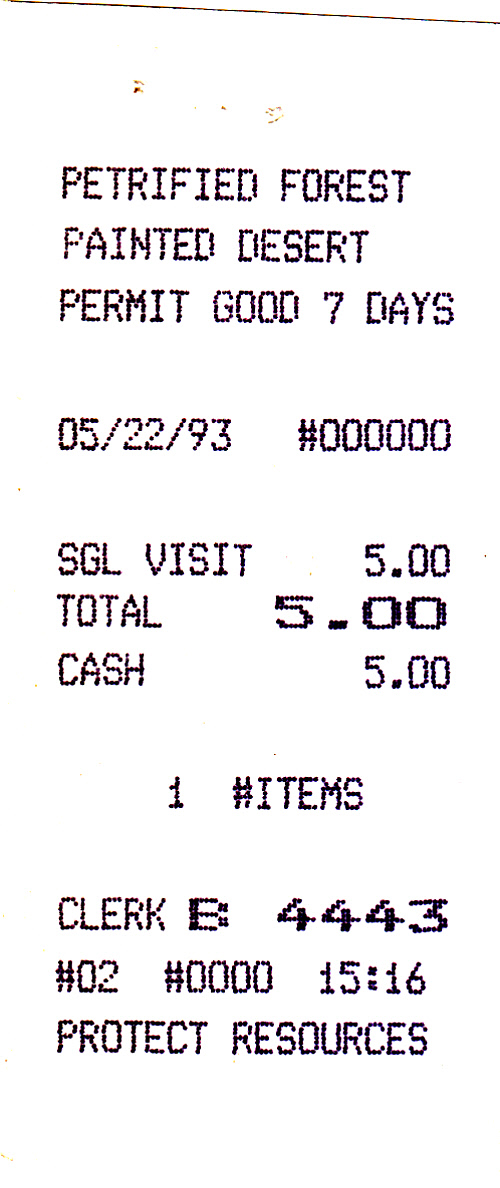This is an image of a receipt printed in block-style dot matrix print, featuring black letters on a white background. At the top, there are noticeable food stains in orange-brown or reddish hues. The top line of text reads "PETRIFIED FOREST" in a dark purple or black font, followed by "PAINTED DESERT" on the next line. Below that, it states "PERMIT GOOD 7 DAYS." The date "05/22/93" is positioned towards the left, while the number "000000" is on the right. The following lines list: "SGL Visit $5.00," "Total $5.00," and "Cash $5.00," with the $5.00 amounts being slightly larger than the other text. Towards the bottom, it reads "1 Items" at the center, and "Clerk B4443" below that. The last lines display "02 000015 16" and the phrase "Protect Resources." There is a prominent black line running across the top of the receipt.